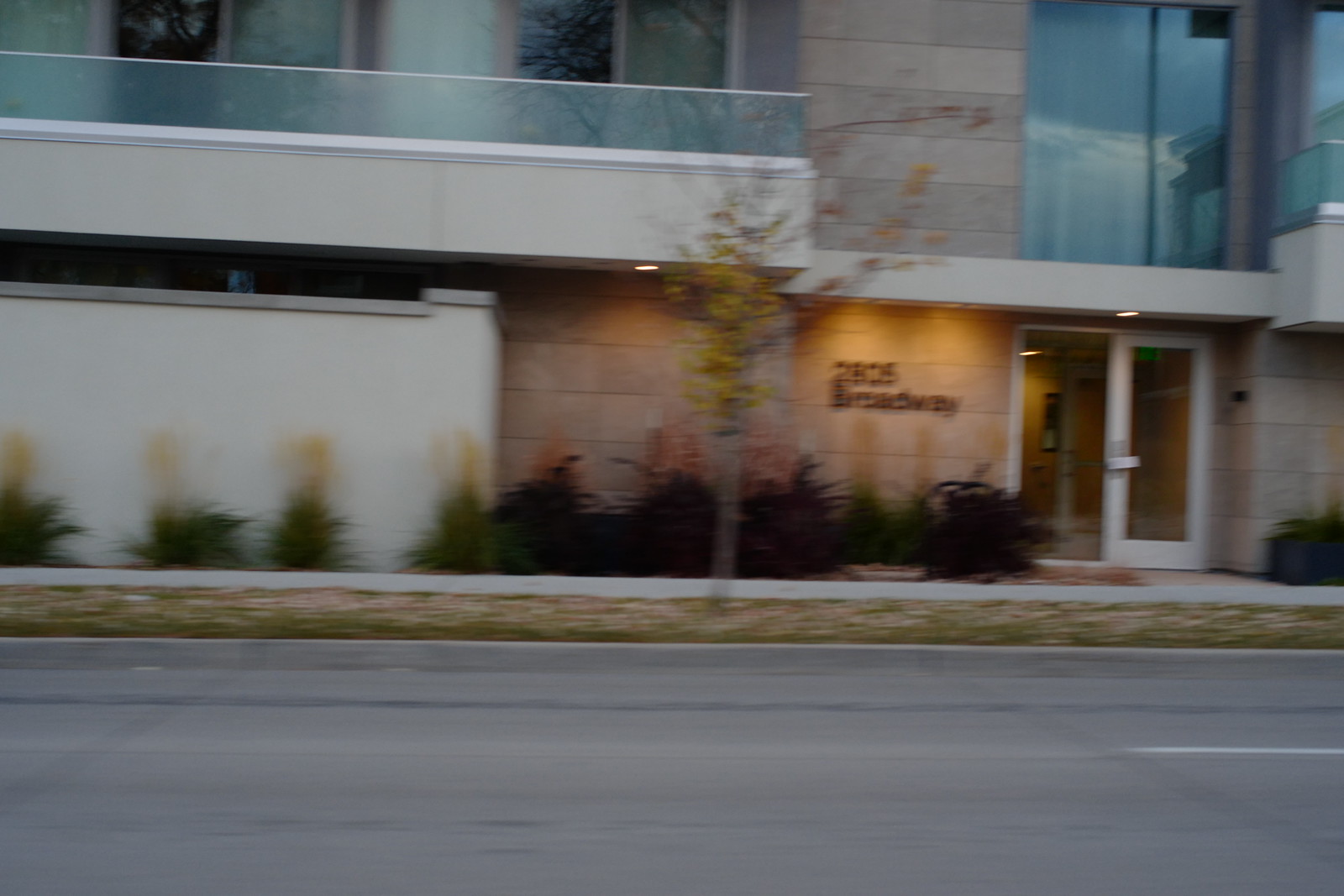The image showcases part of a building, possibly an apartment complex or office space, though its precise purpose remains unclear. The foreground features a street with a white line and curb, adjacent to a stretch of brownish-green grass and a small tree with brown and gold leaves. At the base of the building, there are small bushes and a white area to the left that resembles a patio, bordered by a white wall.

The structure itself is made of brown brick, with glass double doors as the main entrance. To the right, another section of the building displays glass elements and what appears to be a partial balcony. There is a prominent, long balcony distinguished by a gray trim with white edging. Above this balcony, glass doors are visible, potentially serving as double patio doors, suggesting residential apartments with spacious balconies.

The image is cut off to the left of the entrance, but visible large lettering reads "2805" followed by an incomplete word ending in "W-A-Y," which is likely the name of the street.